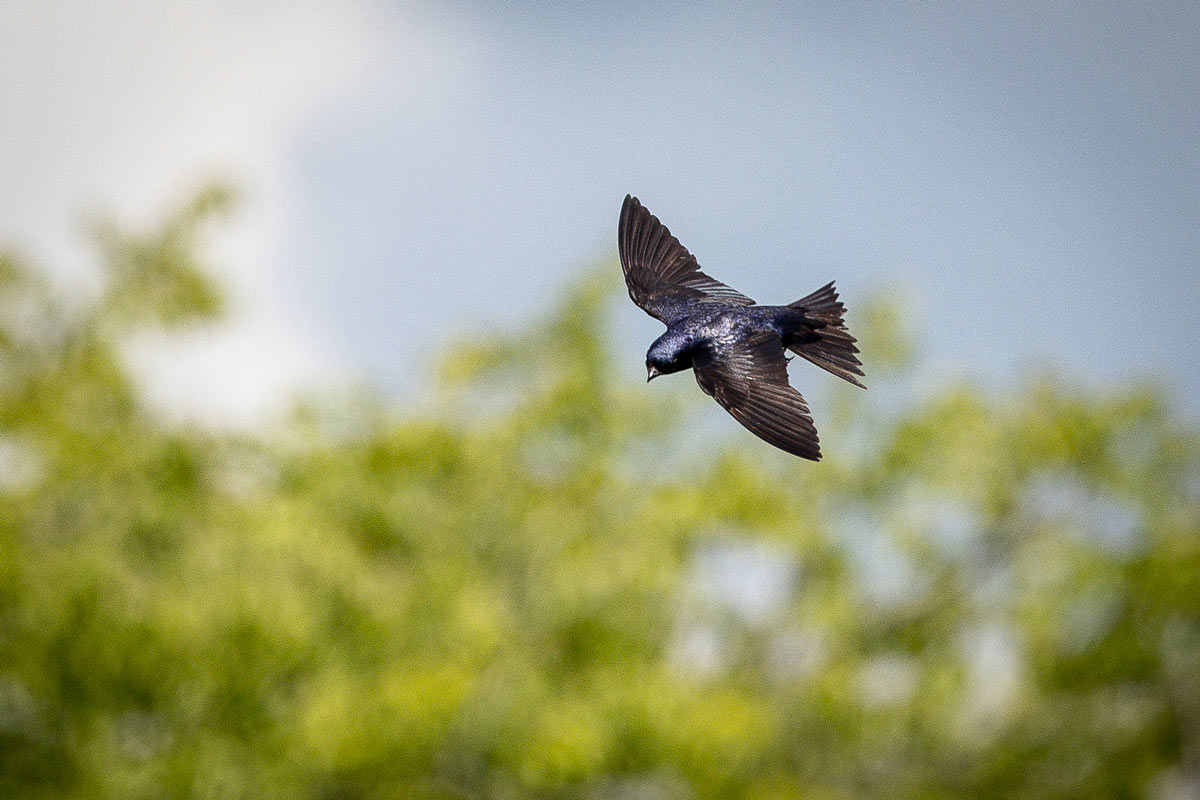The photograph captures a small bird in mid-flight, positioned slightly right of center in the frame. The bird, with its dark blue and black feathers glistening in the sunlight, has its wings fully outstretched, reaching towards both the top and bottom of the frame. Its beak, pointed downwards towards the bottom left corner, gives the impression that it is searching the ground below. The background is a mix of blurry green tree branches occupying the bottom half and a bright blue sky with a single fluffy white cloud in the top left corner. The outdoor setting underlines a sunny day, with subtle details such as shiny feathers on the back of the bird's head and a distinct white patch on its back. The tops of the trees seem to lean slightly to the right, hinting at a gentle wind. This detailed scene beautifully showcases the bird gracefully flying amidst its natural environment.